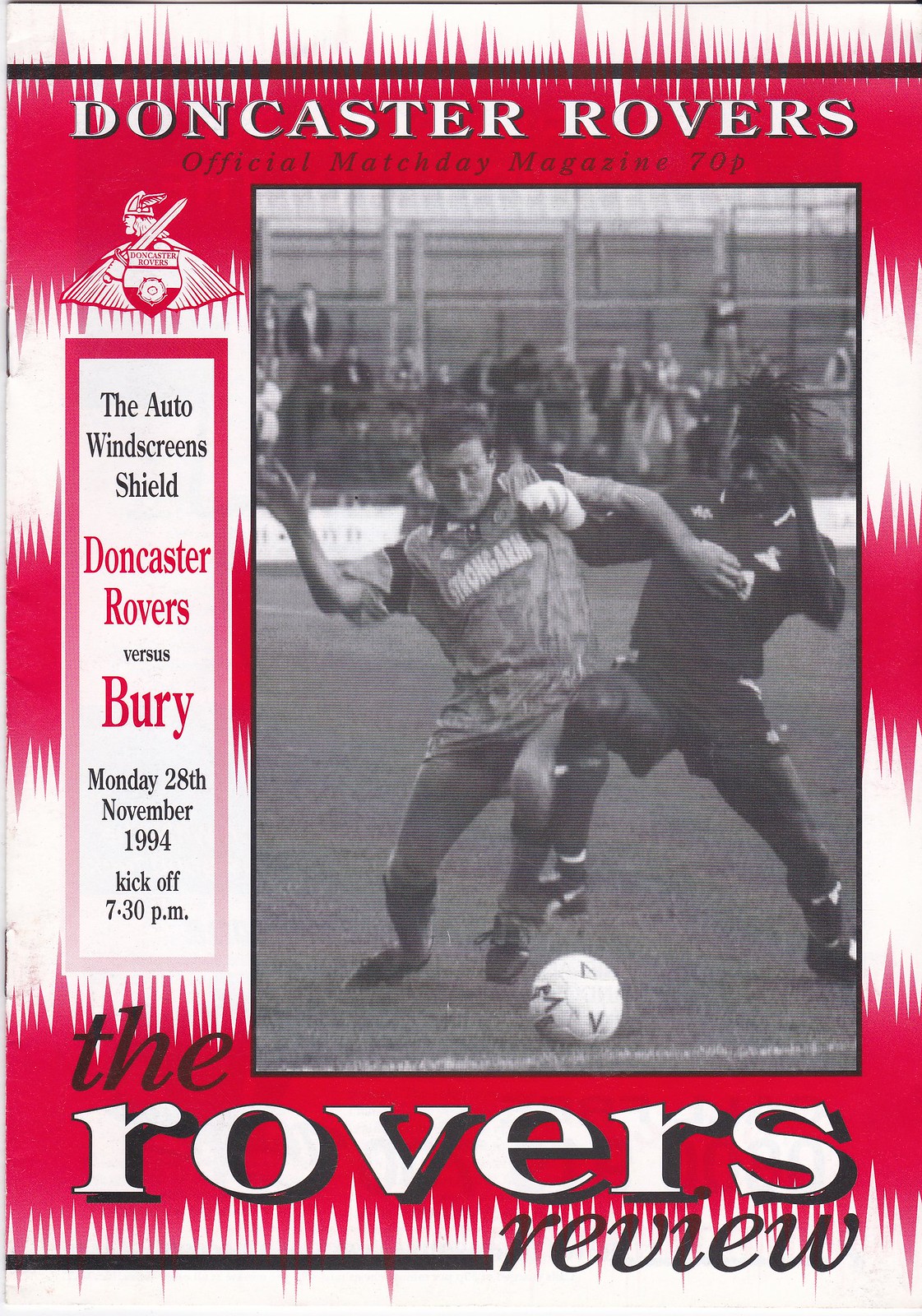The cover of this football game program is the front of the Doncaster Rovers Official Match Day Magazine, priced at 70 pence. It features a red and white static heartbeat-like background pattern with black details. Dominating the center is a large, black and white photograph of an intense soccer match. In the image, an African-American player dressed in dark colors faces off against a Caucasian opponent in a patterned jersey, both poised to kick the soccer ball. The title "Doncaster Rovers Official Match Day Magazine 70P" is prominently displayed across the top, flanked by the team’s emblem featuring a knight. A white box with a red gradient border on the left side announces the Auto Windscreen Shield match between Doncaster Rovers and Bury, scheduled for Monday, the 28th of November, 1994, with kickoff at 7:30 p.m. At the bottom, in large letters, the title “The Rover Review” is showcased, affirming the name of the magazine.